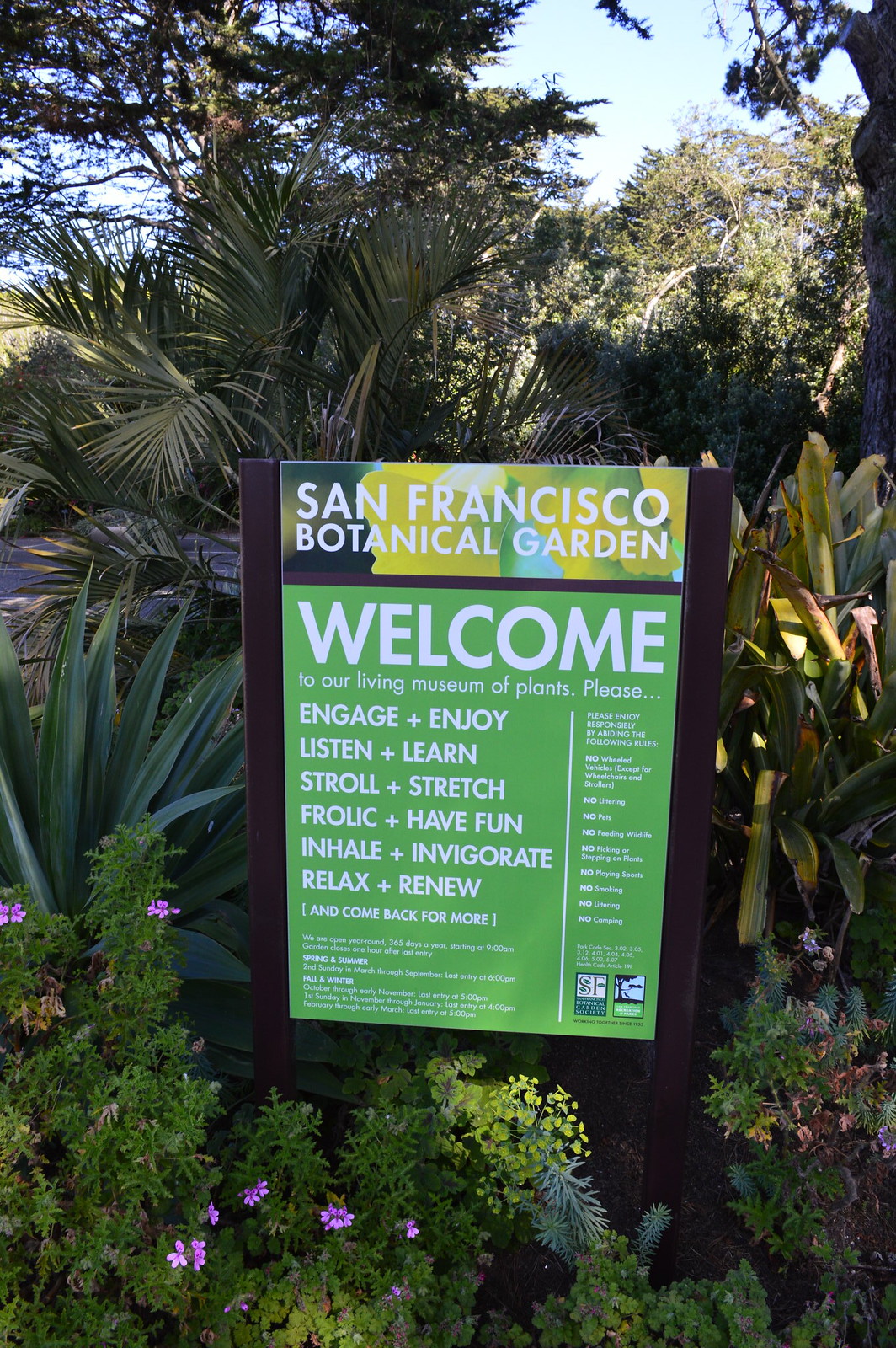This outdoor scene captures a vibrant, lush area abundant with greenery, tropical plants, and trees. The focal point is a sign supported by two dark posts, likely black. At the top, against a yellow floral background, the sign features the text "San Francisco Botanical Garden" in white. Below, a black line separates this title from a green background highlighted with white text that reads: "Welcome to our Living Museum of Plants. Please engage and enjoy, listen and learn, stroll and stretch, frolic and have fun, inhale and invigorate, relax and renew, and come back for more." The rest of the sign includes operational details about the garden being open all year round, with specific seasonal information. Additionally, rules are listed on the right side, indicating no wheeled vehicles, littering, pets, feeding wildlife, picking or stepping on plants, playing sports, smoking, or camping. Two logos appear at the bottom right of the sign, one of which includes the initials "SF." This scene is brightened by a clear blue sky peeking through the dense foliage, while various green plants and purple flowers frame the area around the sign.